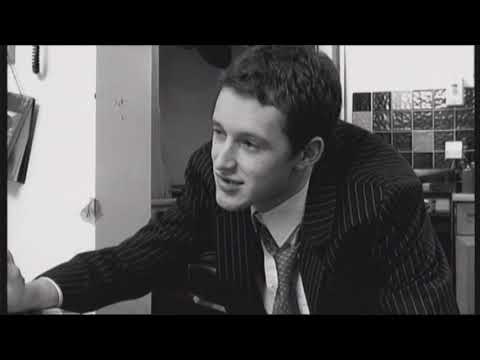This vintage black-and-white photograph captures a lively scene of a family in a cozy, well-lived-in living room. The room is adorned with various personal effects such as pictures on the walls, plants, shelves, and a lamp, hinting at the warm and familiar ambiance of a lived-in home. Central to the image is a couch where an array of family members is either seated or perched on the back edge. From left to right, an older woman, likely the grandmother, is seated next to a little boy who sits in the middle. To the right of the boy is a younger woman, who stands out with her resemblance to a young Janine Garofalo, complete with glasses. Behind the couch, two men, possibly in their middle years, stand or lean with hats worn sideways or backwards, adding an air of casual goofiness to the scene. None of the family members seem to be focusing on the camera, giving the photo a candid feel reminiscent of a moment from a TV sitcom. The playful expressions and lack of direct gaze suggest they might be engaged in a light-hearted moment, perhaps not even aware that their picture was being taken.